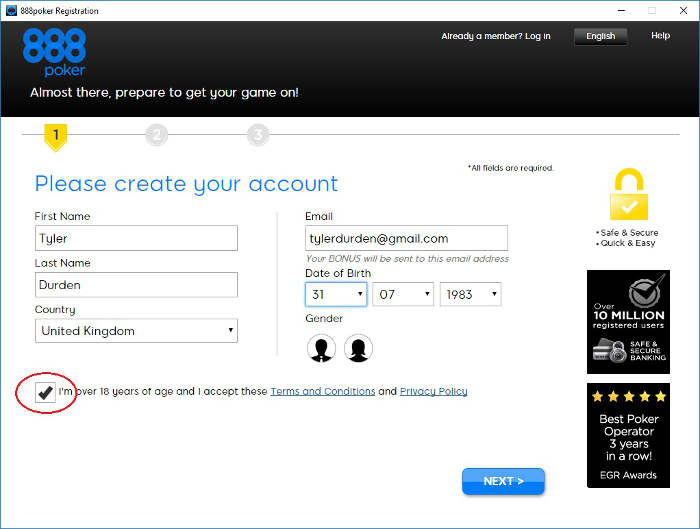This image is a screenshot of a registration page for the service 888Poker, which is presented in a design reminiscent of an old Windows application. At the top of the interface, there is a classic silver bar featuring the typical minimize, maximize, and close buttons arranged from left to right. Displayed in black text on the upper left corner of this bar is the title "888Poker Registration."

Immediately below this title bar, there is a black banner with "888Poker" prominently written in blue text. Just beneath this banner, in white text, the phrase "Almost there, prepare to get your game on" encourages users to proceed with the registration process. The main body of the page is set against a clean white background and consists of numerous fields where users are required to enter their personal details to create an account. These fields include first name, last name, country, email address, and date of birth.

Towards the bottom of the form is a mandatory checkbox accompanied by the statement: "I'm over 18 years of age, and I accept these terms and conditions." This box is checked in the screenshot, and a red circular highlight has been added around this section, presumably to emphasize the importance of this detail in the visual reference.